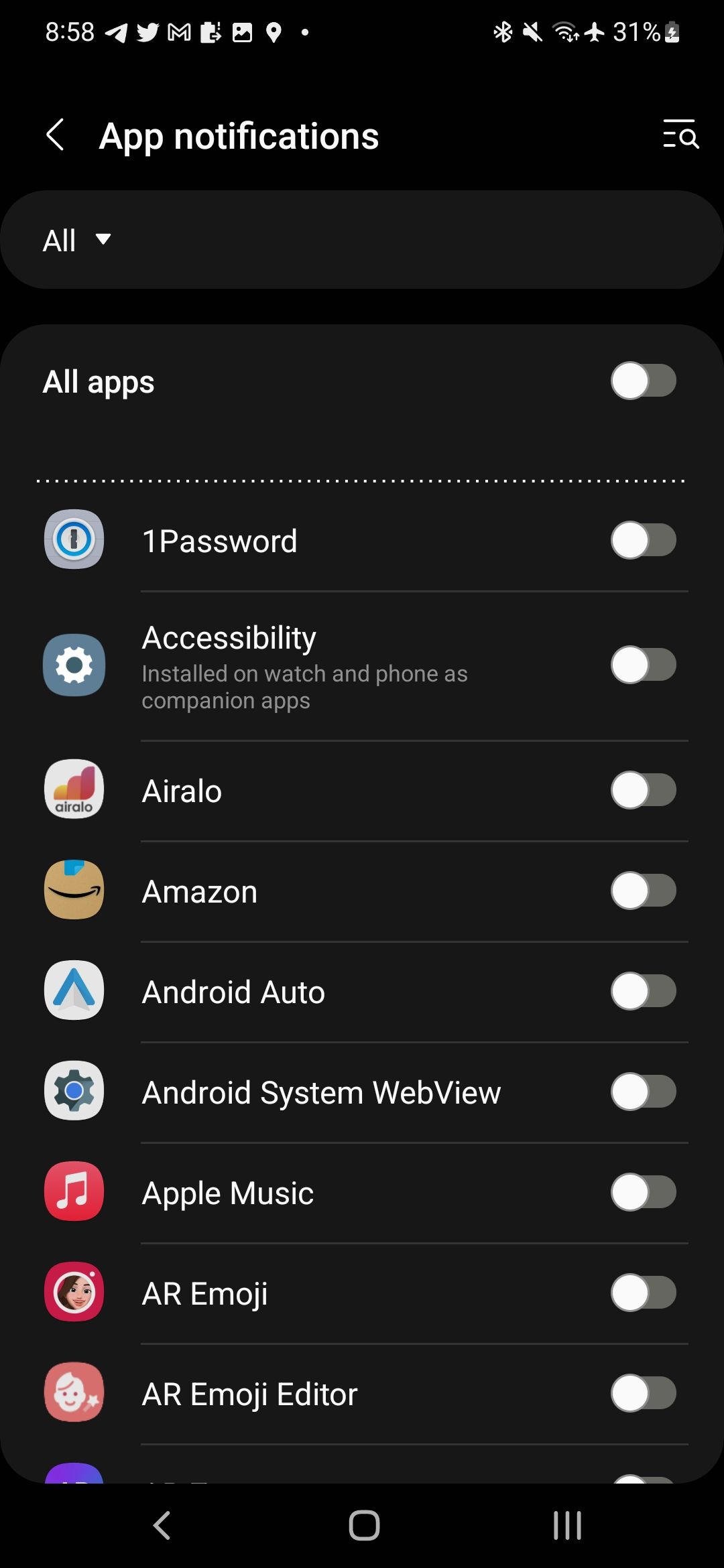This image displays a phone screen with a black background showing the app notification settings page. At the top of the screen, numerous icons are visible, indicating various phone statuses: a Twitter icon, a camera or photo icon, a maps icon, the Bluetooth symbol, a mute button, airplane mode, a Wi-Fi symbol, and remaining battery life at 31% accompanied by a lightning bolt, suggesting the phone is charging. The time displayed is 8:58.

Below these icons, the title "App notifications" is prominently shown. Under this title, there is an "All" button followed by a heading "All apps" accompanied by a toggle switch. All toggle switches in the list are turned off, and the list includes about nine visible items before being cut off at the screen's edge. The items listed are "1Password," "Accessibility" noted as installed on both watch and phone as companion apps, "Aurelio," "Amazon," "Android Auto," "Android System WebView," "Apple Music," "AR Emoji," and "AR Emoji Editor."

At the bottom of the screen, the interface displays the phone's navigation icons: a left-pointing arrow, a rounded square, and three horizontal lines suggesting the home, back, and menu functions.